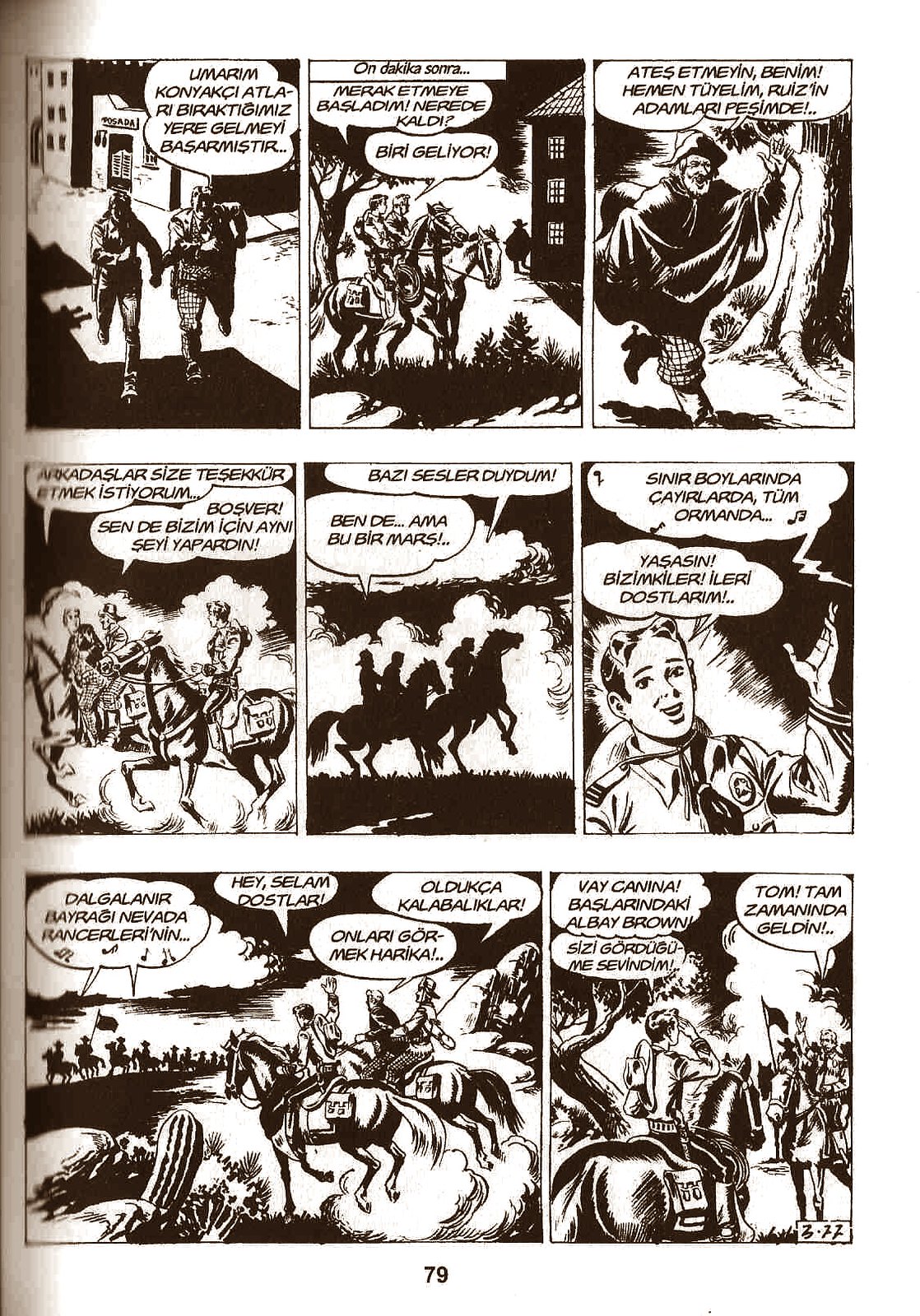This black-and-white comic book page, presumably from an Old West-themed issue, features eight panels showcasing various dynamic scenes. The first panel depicts two figures running, while the second shows a group of men riding on horseback. In the third panel, an old gentleman is seen running and appears to be holding something while yelling. The fourth panel continues with individuals on horseback, seemingly in pursuit of something. The fifth panel presents a dramatic black silhouette of horses, suggesting a nighttime setting. The sixth panel introduces a young boy dressed in a Boy Scout or similar military outfit, speaking emphatically. The seventh and eighth panels, larger than the ones above, illustrate what looks like a battle scene: in the seventh, troops are riding in the background with horsemen to their right, possibly armed, and the young Scout is seen saluting another person on horseback. This page, marked as page 79 and possibly dated either 322 or 327, is intricately detailed, highlighting a moment of intense action and tension.